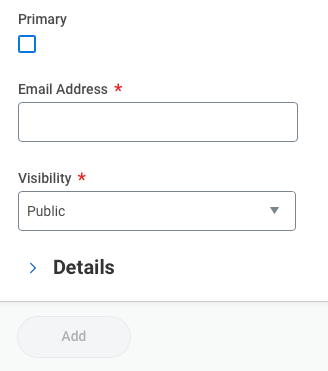The image features a minimalist design on a white background. In the upper left corner, the word "Primary" is displayed in a thin, gray typeface. Below this, a square icon in a vivid navy or royal blue color with a white interior is present. Underneath the square, the text "Email Address" appears in gray, accompanied by a red asterisk indicating a required field. There is a long, empty rectangular text box for inputting an email address.

Further down, the word "Visibility" is also shown in gray with a red asterisk beside it, suggesting it is another mandatory field. Next to this, there is a text box displaying the word "Public" and includes a drop-down menu for selecting other options. A blue arrow pointing to the right is aligned with the bold word "Details".

At the bottom of the image, situated within a gray section of the page, is a gray button labeled "Add" (ADD).